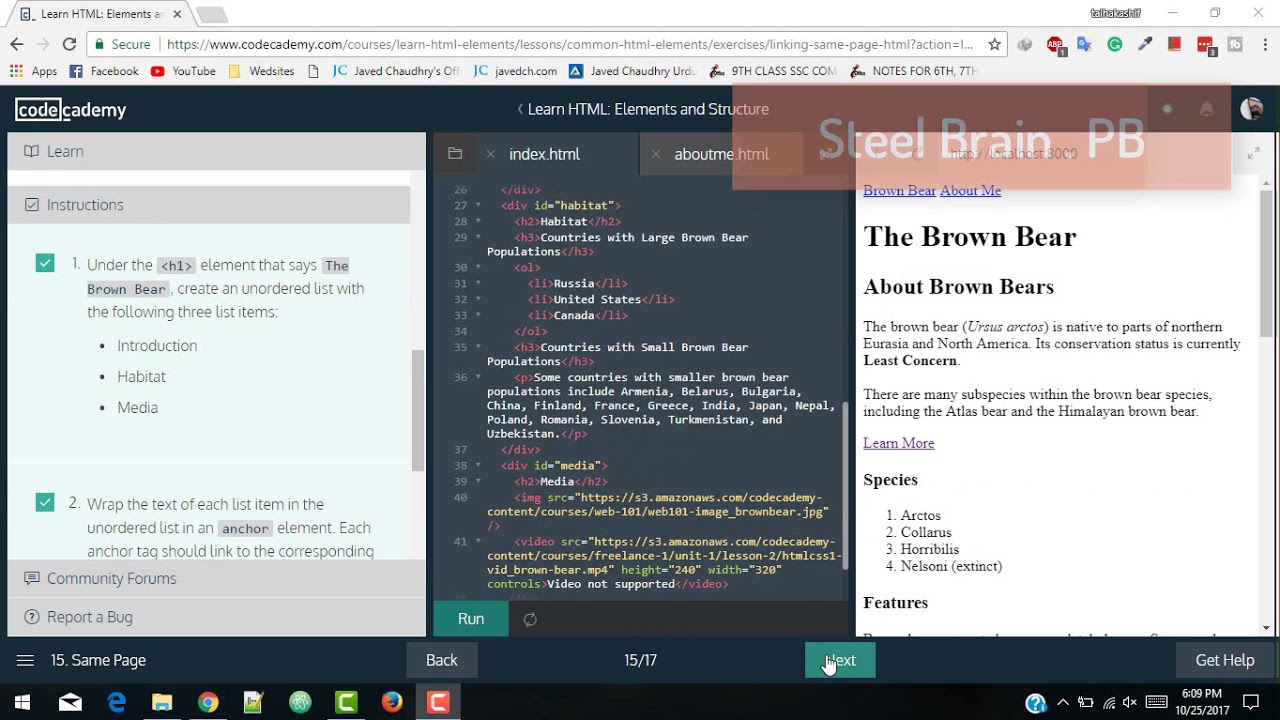This screenshot captures the interface of the Code Academy website. In the upper left corner, the recognizable Code Academy logo is prominently displayed; it features the word "code" encased in a white box, while the rest is written in white lowercase letters against a very dark gray top bar.

The webpage is divided into three distinct sections. 

On the left side, a segment with a white background is topped by a gray bar labeled "Learn," followed by another labeled "Instructions." Below these labels, a set of instructions is clearly visible in white text.

The central panel has a dark gray background and displays lines of HTML code, highlighted in white, yellow, and red for different elements. At the top of this panel, the title "Learn HTML: Elements and Structure" appears in white text.

On the right side, another white background panel contains a section with the headline "The Brown Bear," followed by a subheading "About Brown Bears" and some descriptive text.

The composition of the website efficiently demonstrates an interactive learning environment where the left panel provides guidance, the middle panel allows for coding exercises, and the right panel offers a preview of the resulting webpage.